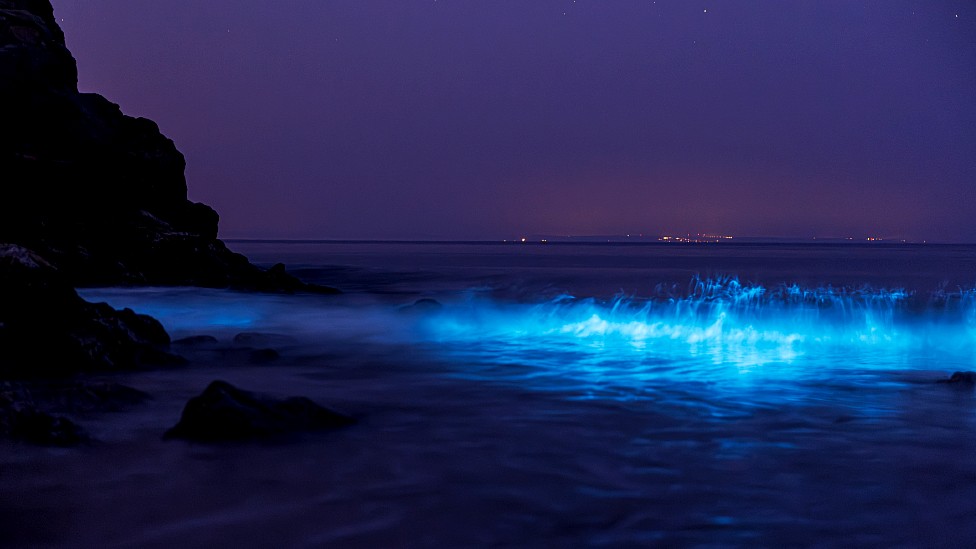In this captivating night scene at the beach, we see a mesmerizing blend of natural and possibly artificial elements. To the left, rugged rock outcroppings stand silhouetted against a dark purple-black sky, while a distant city or town lights up the horizon on the right, casting a faint glow in the background. The photograph's most striking feature is the wave breaking at the forefront, illuminated by a brilliant neon blue bioluminescence that almost appears otherworldly. This glowing wave creates a stark contrast against the shadowy textures of the ocean and beach, making the entire scene look surreal and enchanting. The light from the distant city and the radiant, almost ethereal blue of the wave together create a breathtaking tableau that captures the mystery and beauty of the night ocean.